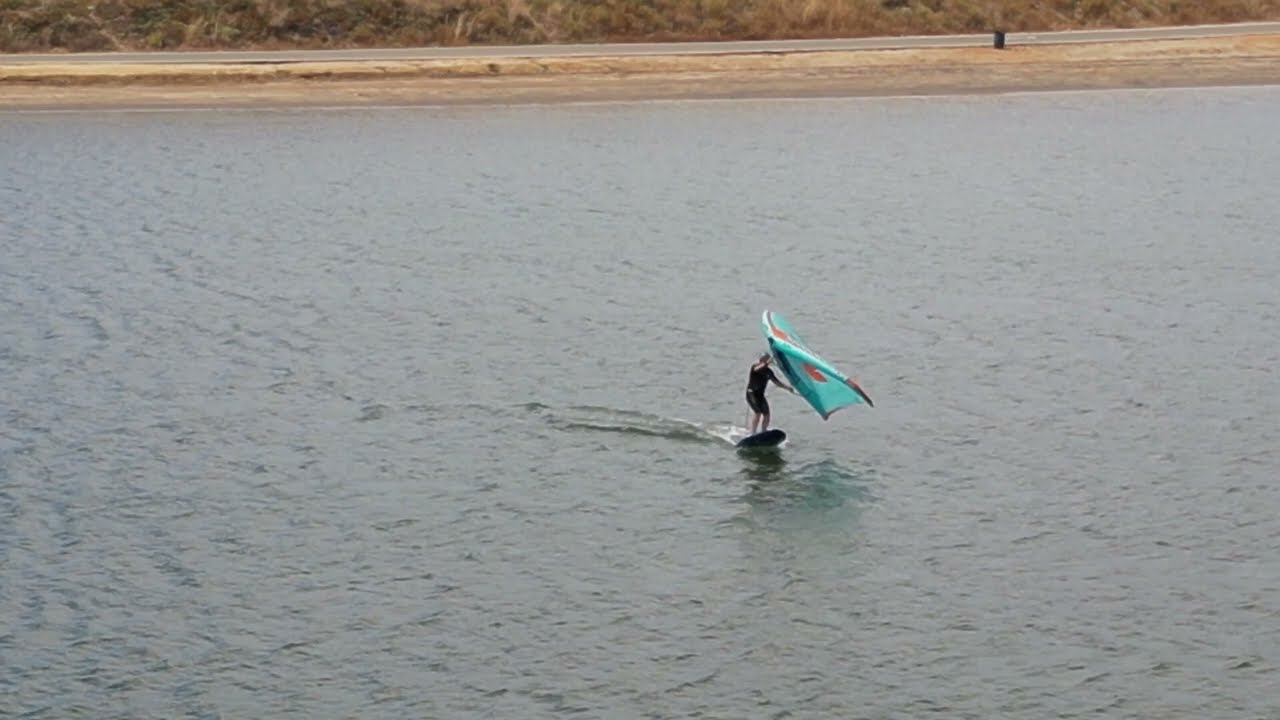The image captures a serene scene of a body of calm water, featuring a solitary figure on a paddleboard or windsurf board. The person, clad in black knee-length shorts and a black long-sleeve top, stands confidently in the middle of the water. They hold a large teal and orange sail above them, suggesting they might be engaging in windsurfing. The board tilts up slightly as they maneuver. A slight wake curves behind the board, accentuating the peaceful, unruffled water surface. In the background, a narrow beach of sand gives way to a single lane road lined with dry vegetation and a solitary bin. The landscape adds a tranquil touch to the overall composition, emphasizing the solitary and focused activity of the individual on the water.